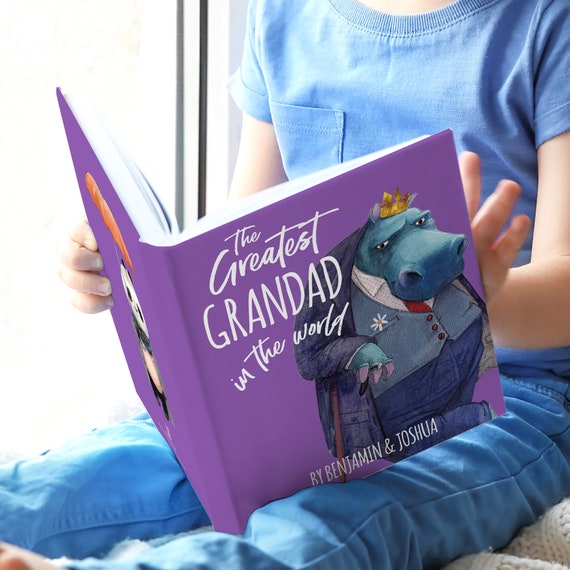In the photograph, a child, dressed in a blue short-sleeve t-shirt with a pocket on the right side and blue jeans, is sitting on the right side of the image, visible from shoulders to knees. The child is intently reading a book titled "The Greatest Granddad in the World" by Benjamin and Joshua. The book has a purple cover with the title and authors' names written in white font. The cover illustration features an anthropomorphic hippopotamus dressed in a three-piece suit, including a white check shirt, red tie, grey waistcoat with red buttons, blue jacket, and jeans. The hippopotamus is depicted wearing a crown and fingerless gloves, leaning on a cane, and holding a daisy with a yellow center. Although the back of the book is not clearly visible, it appears to display a panda image, possibly a logo. The child holds the book with both hands, with fingers curved around the left side and splayed on the right side, as if in the act of turning a page. This detailed scene creates a vivid depiction of the advertisement for "The Greatest Granddad in the World," capturing the whimsical art and engaging narrative that the book promises to deliver.